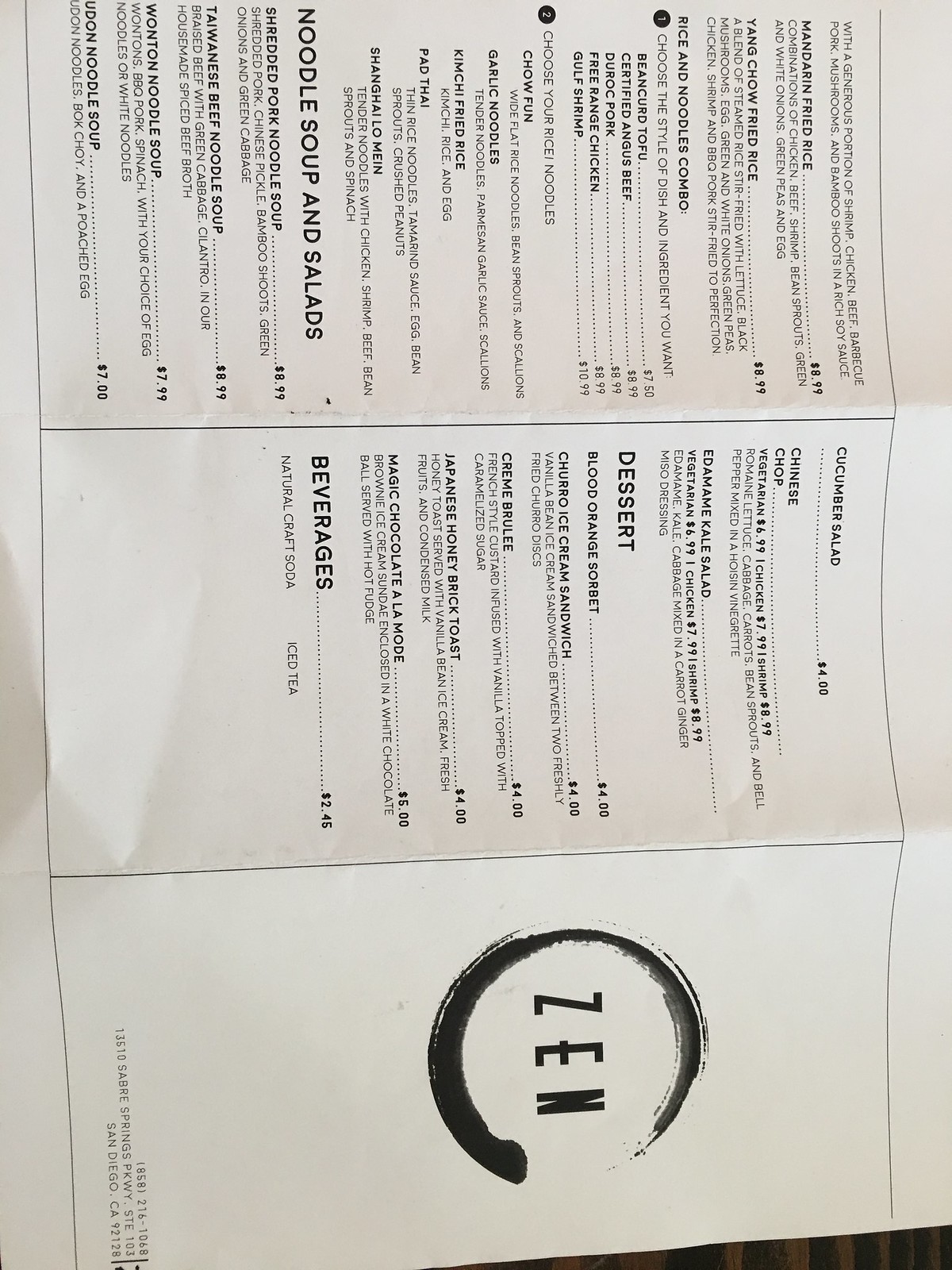The image features a sideways view of a menu titled "Zen," with the word "Zen" oriented vertically, as if aiming downward. The menu is white with black print and includes a distinctive circular diagram – a thick black circle that tapers into a thinner line – encircling the "Zen" text. The menu items are partially visible and include a section for desserts with an entry for something involving blood orange, though the full details are hard to discern due to the small text size. 

Below, there is a beverages section listing an item priced at $2.46 and what seems to be craft soda. There's also a mention of cucumber salad, possibly priced around $4, though the figure is not entirely clear. The main course section includes dishes such as mandarin fried rice and yang chow fried rice. At the bottom of the image, the menu rests on a surface resembling wood grain, featuring alternating dark brown and light brown patterns.

Additionally, there are headings for noodle soups and salads, indicating the variety of offerings, but part of the menu remains out of frame, leaving some items out of view.